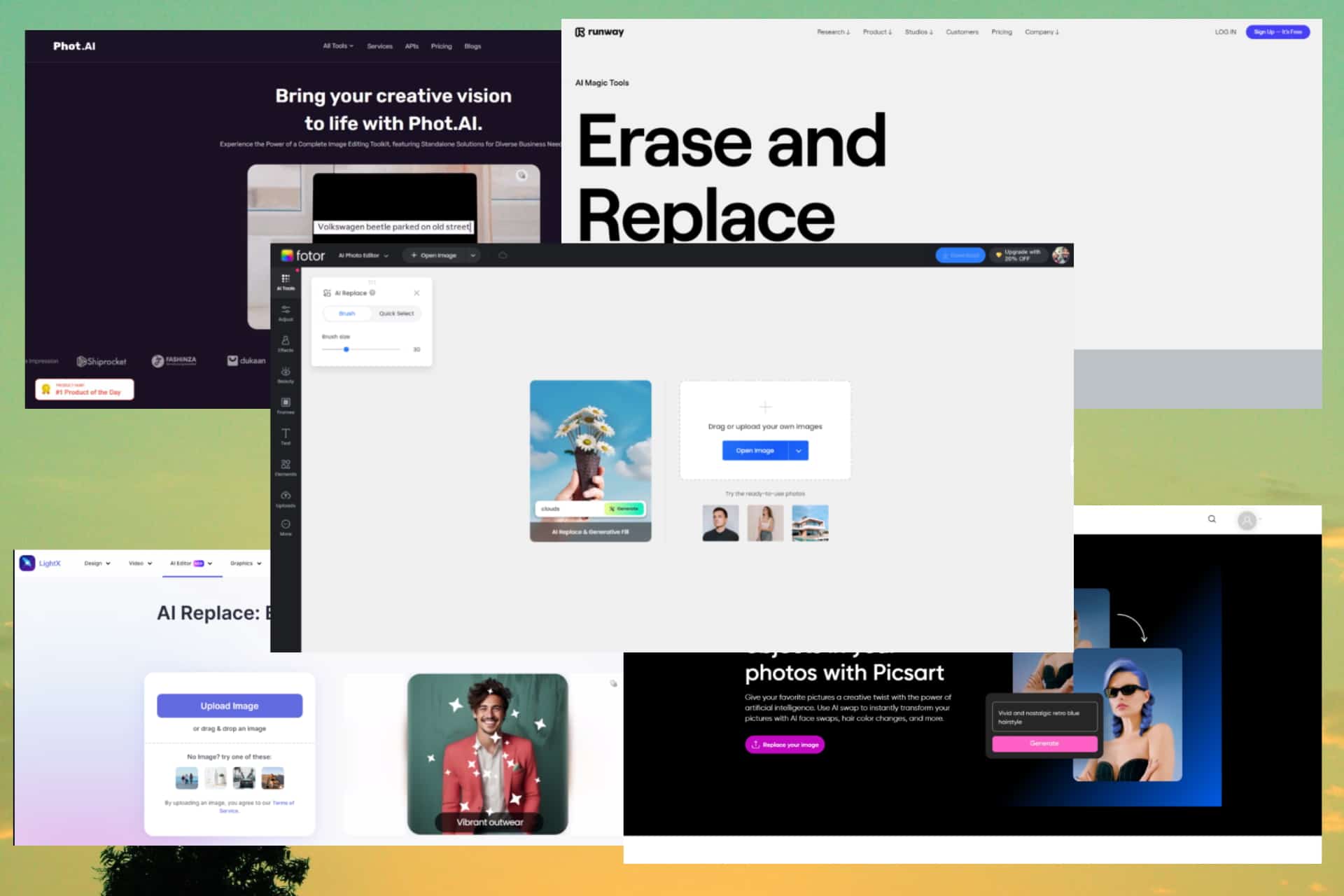The image showcases a digital workspace dedicated to photo AI creation. The backdrop features a black interface filled with several overlapping boxes, each representing different tools and functionalities of the photo AI platform.

In the most prominent box, the text "Phot.ai, bring your creative vision to life with Phot.ai" is displayed over a black background. Overlaying this is the phrase "Volkswagen Beetle parked on an old street," suggesting an example image that the AI can generate or manipulate. At the center, another box labeled "Photor" invites users to drag or upload their images into the platform, indicating an interactive interface.

Above this central box, a banner reads "Erase and Replace" accompanied by another box labeled "AI Magic Tools - Run Away." Below these, there is another prominent section marked "Photo with Pixart," and within this box, several directional arrows point towards an image of a woman with strikingly blue hair, showcasing the AI's capability to wildly alter photo elements.

Further down, the "AI Replace" section stands out with an upload prompt set in white text against a purple background. Here, an image features a man wearing a salmon-colored jacket and a white collared shirt, standing under a virtual sky filled with stars. The man has dark hair, a mustache, and a welcoming smile. 

Underlying the entire interface is a surreal background painted in hues of green and orange, hinting at a scenic sky with a faint silhouette of a tree at the bottom left, adding an artistic touch to the technologically advanced workspace.